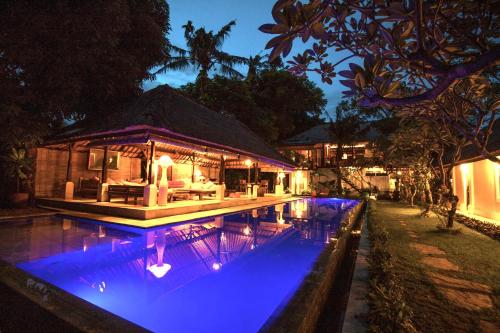In the early evening light, this enchanting scene captures what appears to be a luxurious backyard, possibly part of a vacation rental. The sky, transitioning to a deeper blue as the sun sets, frames a serene and welcoming atmosphere. Central to the setting is a long, rectangular swimming pool, lit from below in a vibrant electric blue, reflecting the surrounding beauty.

On the left side of the image, a charming, open shelter with a Caribbean-esque feel is visible. This structure, adorned with warm, inviting lights, features comfortable furniture and possibly a grill, suggesting a perfect spot for relaxation or social gatherings. To its right, a stone patio leads towards the main house, which spans the back and right side of the image. While the house is partially obscured by a lush array of tall palm trees and vivid green foliage, its welcoming glow emanates through the trees, highlighting the pathway and patios.

The house itself appears to be a one-story building with a hipped roof, accented by outdoor furniture and softly glowing lamps. The entirety of the scene is enhanced by the interplay of light and reflections in the pool, creating a tranquil yet vibrant setting that beautifully merges natural and architectural design elements.